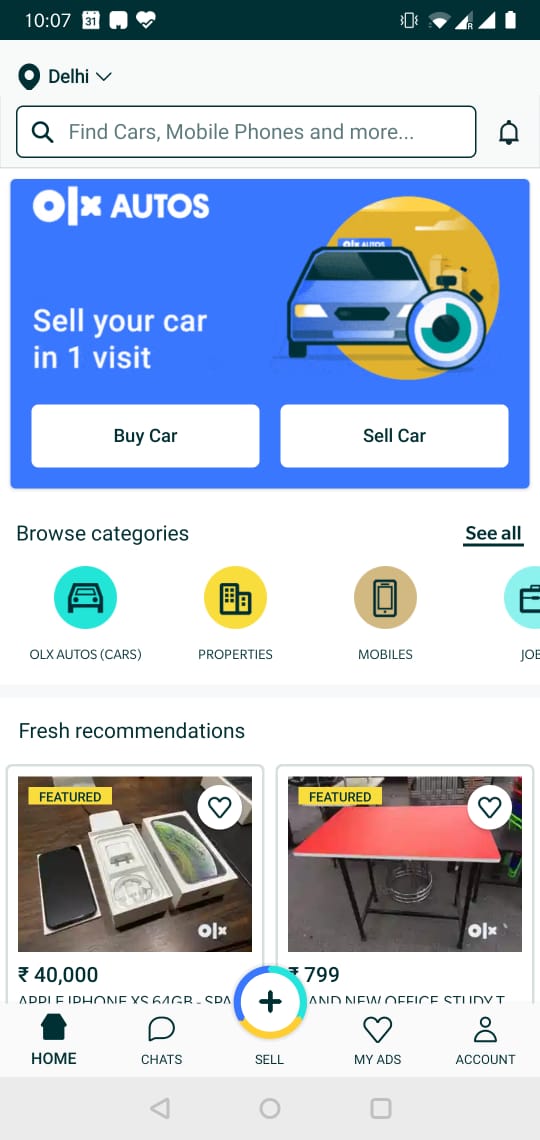This screenshot showcases the interface of a selling app, likely targeted towards users in India, as indicated by the "Delhi" location displayed at the top-left corner. Directly beneath the location label is a search bar, enabling users to input search terms to navigate the website. Below the search bar, an advertisement for 'OX Autos' is prominently positioned. Following the ad, there is a horizontal scrolling 'Browse Categories' bar, allowing users to explore various product categories. Further down, the 'Fresh Recommendations' section highlights featured products, currently showing an Apple iPhone XS and a Red Office Desk. The layout is designed to facilitate easy navigation and discovery of products for sale.